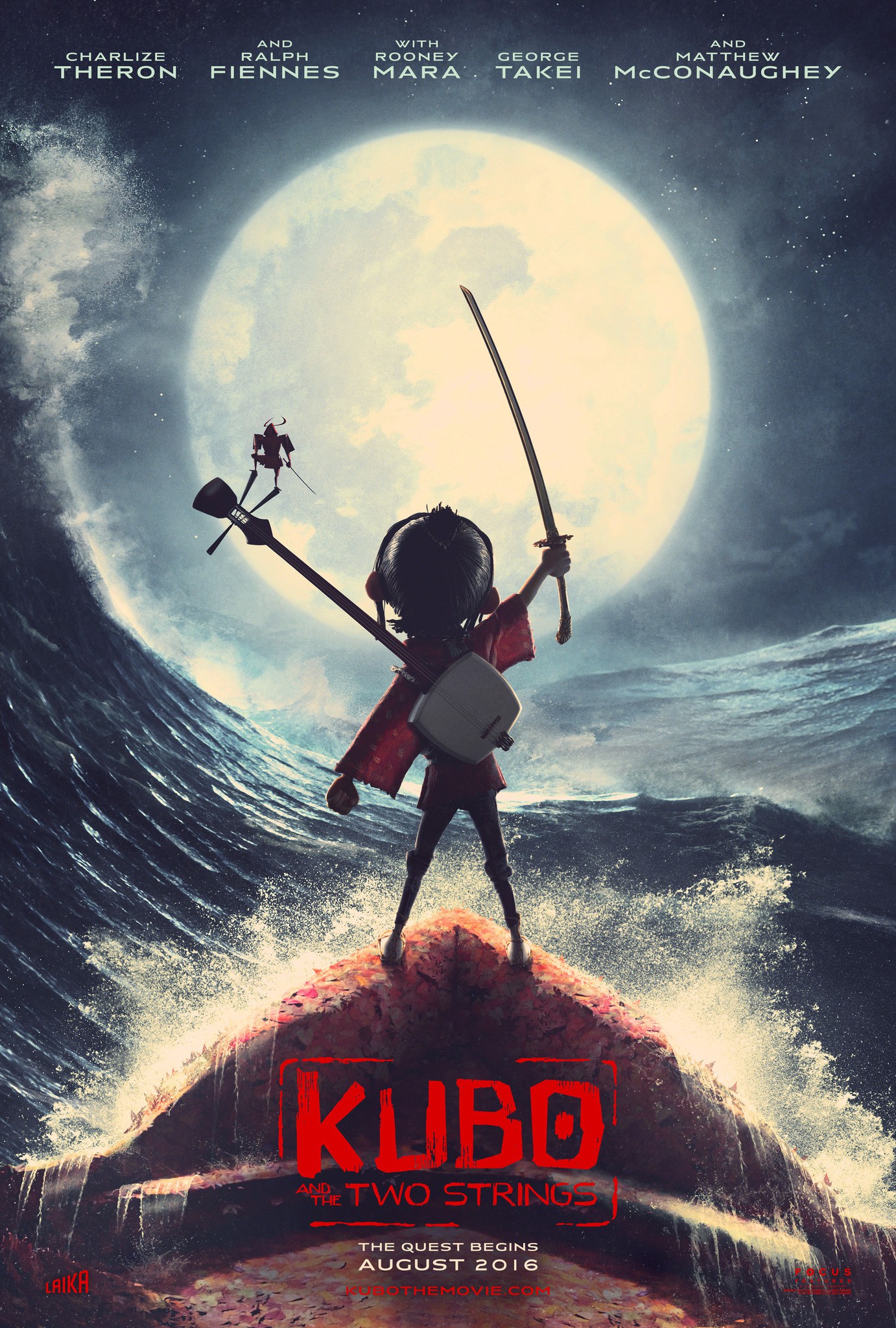This detailed movie poster illustration for "Kubo and the Two Strings" features a young boy, presumably Kubo, standing boldly in a red kimono with a distinctive white stringed instrument slung across his back. He holds a katana aloft with determination, aiming it towards a prominent full moon that dominates the night sky behind him. The moonlight casts a dramatic silhouette of Kubo, who is positioned on the fo’c’sle of a boat navigating rough seas; a sizeable tidal wave curves in harmony with the moon’s shape, adding a sense of impending adventure and peril. Notably, a small figure resembling a Viking with a horned helmet stands on the end of Kubo's guitar, adding a whimsical touch. The poster’s title, "Kubo and the Two Strings," appears at the bottom in bold, scratchy red paintbrush strokes, with the tagline "The quest begins August 2016" below. Additionally, the prominently displayed names of the starring actors—Charlize Theron, Ralph Fiennes, Rooney Mara, George Takei, and Matthew McConaughey—are listed at the top, setting the stage for an epic cinematic journey.